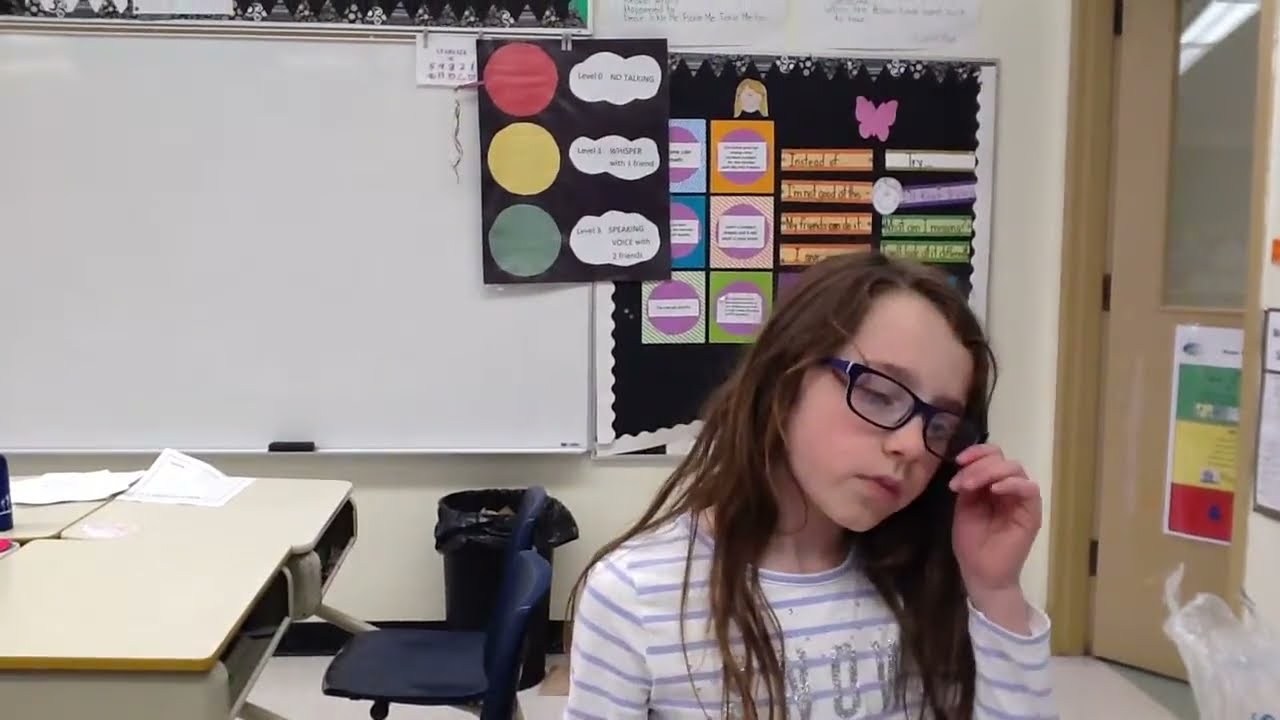The photograph captures a young girl in an elementary school classroom. She is Caucasian with fairly pale skin and long, somewhat straggly brown hair. The girl is wearing black glasses, which appear slightly crooked as she adjusts them with her left hand. Her left eye is closed while the right eye remains open, indicating she might be fiddling with her eyesight. Her attire includes a long-sleeved white shirt featuring light lavender horizontal stripes and partially obscured silver, sparkly lettering on the front. 

The classroom setting around her is detailed and vivid. Behind her to the left is a large whiteboard, with a blue swivel chair and a black bin beneath it. To the right of the whiteboard is a black poster board adorned with various colorful notices and small posters, including a prominent traffic light symbol with words like "level zero, no talking," “level one, whisper with a friend," and "level three, speaking voice with two friends." Additionally, a purple butterfly outline is visible in the upper right corner of this black board. 

In the foreground, there are a couple of school desks with black seats, and a wooden door with a window at the top is slightly open, revealing a hallway lit by a fluorescent tube light. A safety sign in green, yellow, and red is placed at the bottom of the door. The girl stands near one of these desks, giving the sense that she has just left her seat. Despite the somewhat dejected look on her face, her presence and the intricate classroom backdrop make for a very engaging image.